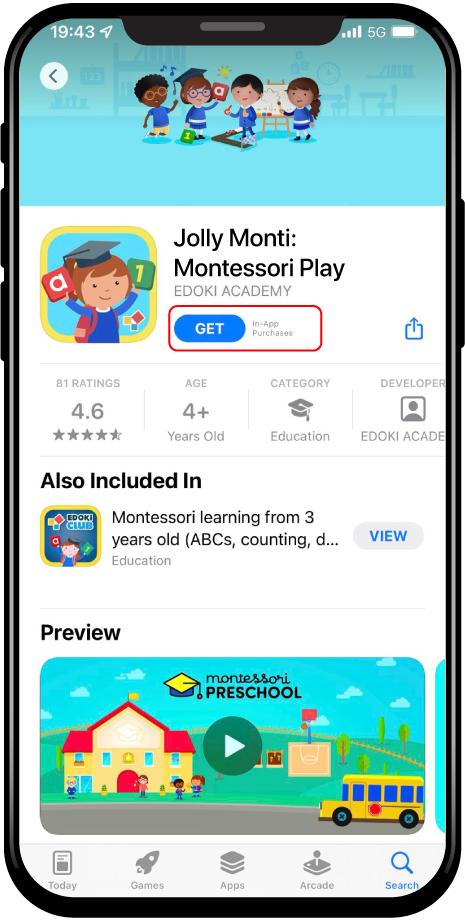In this image, we see a black cell phone with its screen turned on. The phone features three buttons on the left side: a short one at the top and two longer ones of equal size situated below it. There is also a long black button on the right side of the cell phone. The screen displays an illustration of four children set against a light blue background at the top. Below this illustration, information about an app called "Jolly Monty Montessori Play" by Idoki Academy is presented. An illustration of a young child wearing a black graduation cap accompanies this text. Further down the screen, there is a red-outlined action button labeled "Get." Below this button, additional app details are provided, including 81 ratings with an average of 4.6 stars, an age suitability of 4+ years, its category as Education, and the developer's name, Idoki Academy. The app is also mentioned to be a part of the "Montessori Learning for Three-Year-Olds" program.